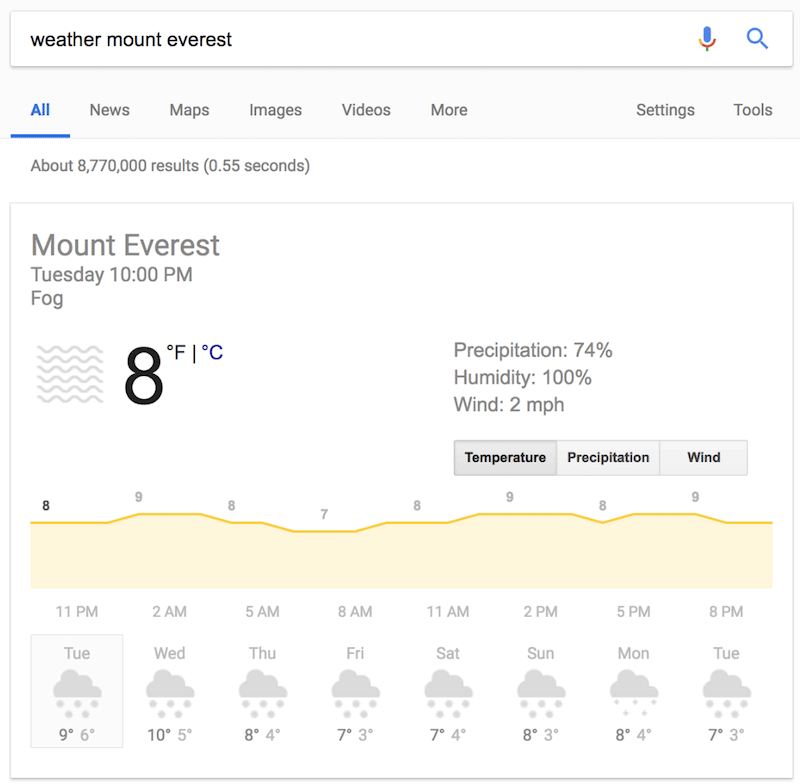The image is a detailed screen capture of a Google search results page focused on the weather in Mount Everest. The search query and results are displayed within a standard Google interface, featuring a black and white address bar at the top. The search term "weather Mount Everest" is clearly visible with a corresponding blue, gold, and red microphone icon, and a blue magnifying glass signifying the search function.

Below this, the page layout shows the categories: All, News, Maps, Images, Videos, More, Settings, and Tools, with the "All" category highlighted by a blue underline. The search results indicate approximately 8,770,000 results retrieved in 0.55 seconds.

The weather details for Mount Everest are provided prominently. At 10 PM on Tuesday, the weather is foggy with the temperature at 8 degrees Fahrenheit, also shown in Celsius. There are icons indicating a 74% precipitation chance, 100% humidity, and 2 MPH wind speed. 

Further down, the weather forecast is illustrated in a graph format with three gray boxes labeled Temperature, Precipitation, and Wind. Orange-colored graphs depict these metrics over time intervals of 11 PM, 2 AM, 5 AM, 8 AM, 11 AM, 2 PM, 5 PM, and 8 PM. The forecast extends from Tuesday through to the following Tuesday. Each day in the forecast shows temperatures and weather conditions, symbolized by cloud icons with water droplets indicating precipitation.

- Tuesday: High of 9°F, Low of 6°F.
- Wednesday: High of 10°F, Low of 5°F.
- Thursday: High of 8°F, Low of 4°F.
- Friday: High of 7°F, Low of 3°F.
- Saturday: High of 7°F, Low of 4°F.
- Sunday: High of 8°F, Low of 3°F.
- Monday: High of 8°F, Low of 4°F.
- Tuesday: High of 7°F, Low of 3°F.

The image ends here with no additional details of note.